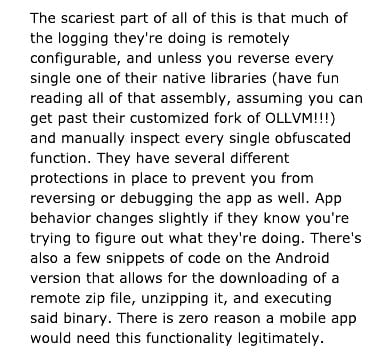The image features a stark white background with black text that reads from top to bottom: "The scariest part of all of this is that much of the logging they're doing is remotely configurable. Unless you reverse every single one of their native libraries, have fun reading all of that assembly, assuming you can get past the customized fork of OLLVM and manually inspect every single obfuscated function. They have several different protections in place to prevent you from reversing or debugging the app as well. App behavior changes slightly if they know you're trying to figure out what they're doing. There are also a few snippets of code on the Android version that allow for the downloading of a remote zip file, unzipping it, and executing said binary. There is zero reason a mobile app would need this functionality legitimately." Below this comprehensive explanation, the remainder of the image is filled with empty white space extending to the bottom edge.